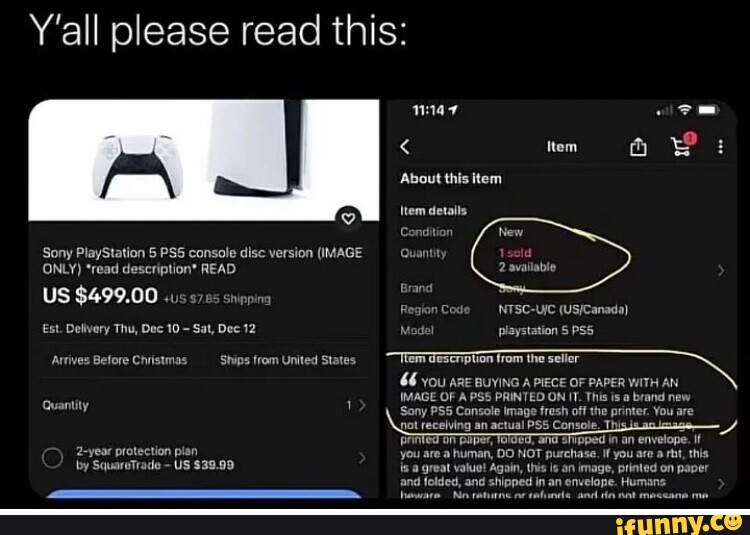This meme, sourced from iFunny.co, features a humorous yet cautionary take on online shopping scams. Set against a black background with white text, the meme begins with a bold plea: "Y'all please read this." It consists of two parts—a fake advertisement and a detailed product description.

On the left, there's a screenshot of an apparent ad for a "Sony PlayStation 5 PS5 Console Disc Version," displayed with a prominent image of the coveted gaming console. Key details of the listing include a suspiciously low price of $4.99, in addition to $7.85 for shipping. The ad emphasizes that the product will arrive between December 10th and 12th, perfect timing for holiday shoppers. Additional information highlights a two-year protection plan available for $39.99.

On the right, the product description reveals the true nature of the listing in a hilariously deceptive fashion. It states that buyers are actually purchasing "a piece of paper with an image of a PS5 printed on it," and not a physical console. The description is loaded with warnings such as "You are not receiving an actual PS5 console," and insists that only robots should proceed with the purchase, humorously cautioning humans against buying the item. The seller makes it clear that the paper image of the PS5 is "fresh off the printer," and further underlines the no-return policy, advising potential buyers not to message them.

All in all, this meme serves as a comedic reminder to read product descriptions carefully to avoid falling for online scams.